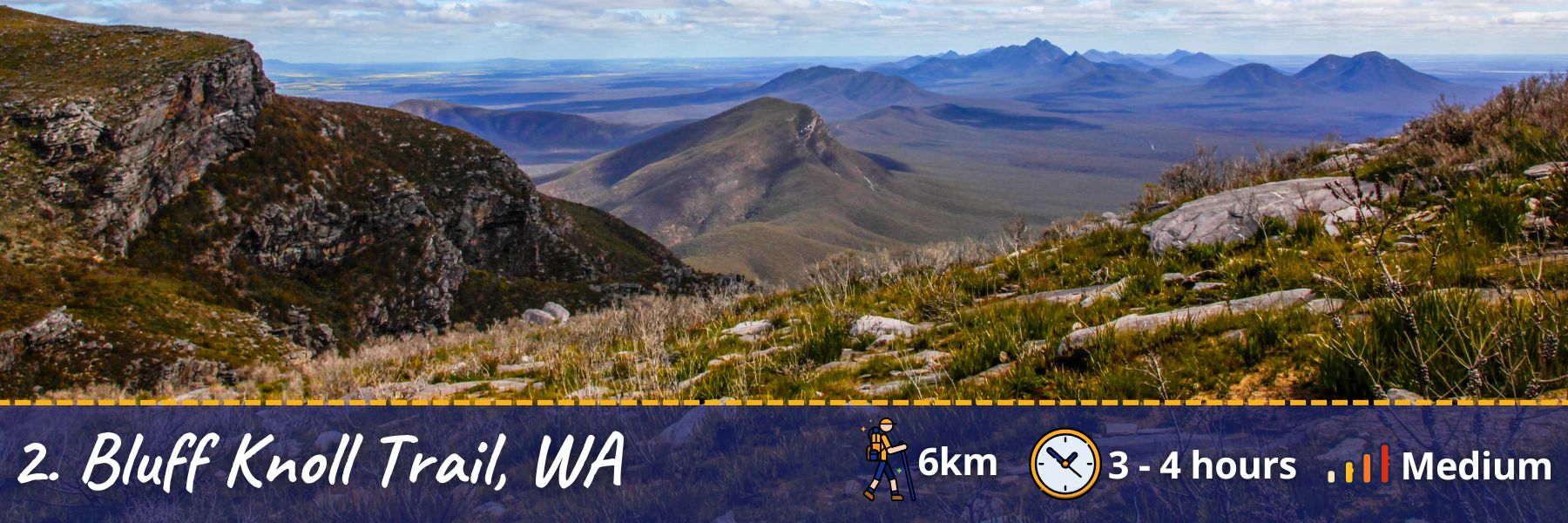This image is a wide, horizontally aligned poster of the Bluff Knoll Trail in Washington, showcasing detailed trail information and scenic elements. The bottom section features a dark blue rectangular area with the number "2" in white, indicating the trail number. It reads "Bluff Knoll Trail, WA" with a trail length of "6 kilometers," an estimated hiking time of "three to four hours," and a "medium" difficulty level. The main image depicts the trail surrounded by shorter trees, grassy areas, and rocks, creating a gently hilly terrain. The left-hand side shows a taller, rocky hill with abundant moss and grass. The background features additional rocky hills and a body of water, possibly the ocean or a lake, under a sky that is a mix of gray clouds and patches of blue. The left side of the image includes the side of a brown and green cliff, while the right side has larger rocks, trees, and grass, descending slightly towards the left. Feedback you’ll find touches on the attractiveness of the setting, suggesting it's an inviting place for a moderate-level hike amidst varied natural landscapes.